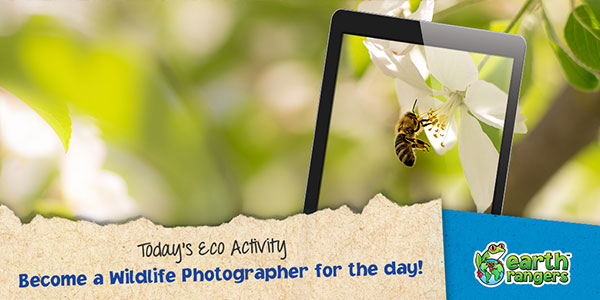This is a rectangular online advertisement for the Earth Rangers app. Dominating the center is an image of a tablet seamlessly blending with the out-of-focus background of flowers and greenery. On the tablet screen, there is a close-up, color photograph of a bumblebee collecting nectar from the petals of a flower. The edges of the image on the tablet align perfectly with the blurred background, enhancing the illusion of a unified scene.

At the bottom left of the advertisement, there is a graphic resembling a ripped piece of paper with black text reading "Today's Eco Activity." Below this, in blue text, it says, "Become a Wildlife Photographer for the Day." On the bottom right, the Earth Rangers logo is displayed in green, featuring a cartoon-style tree frog sitting atop the Earth. The overall design suggests that the Earth Rangers app encourages users, possibly children or nature enthusiasts, to engage in environmental discovery and photography activities using their mobile devices.